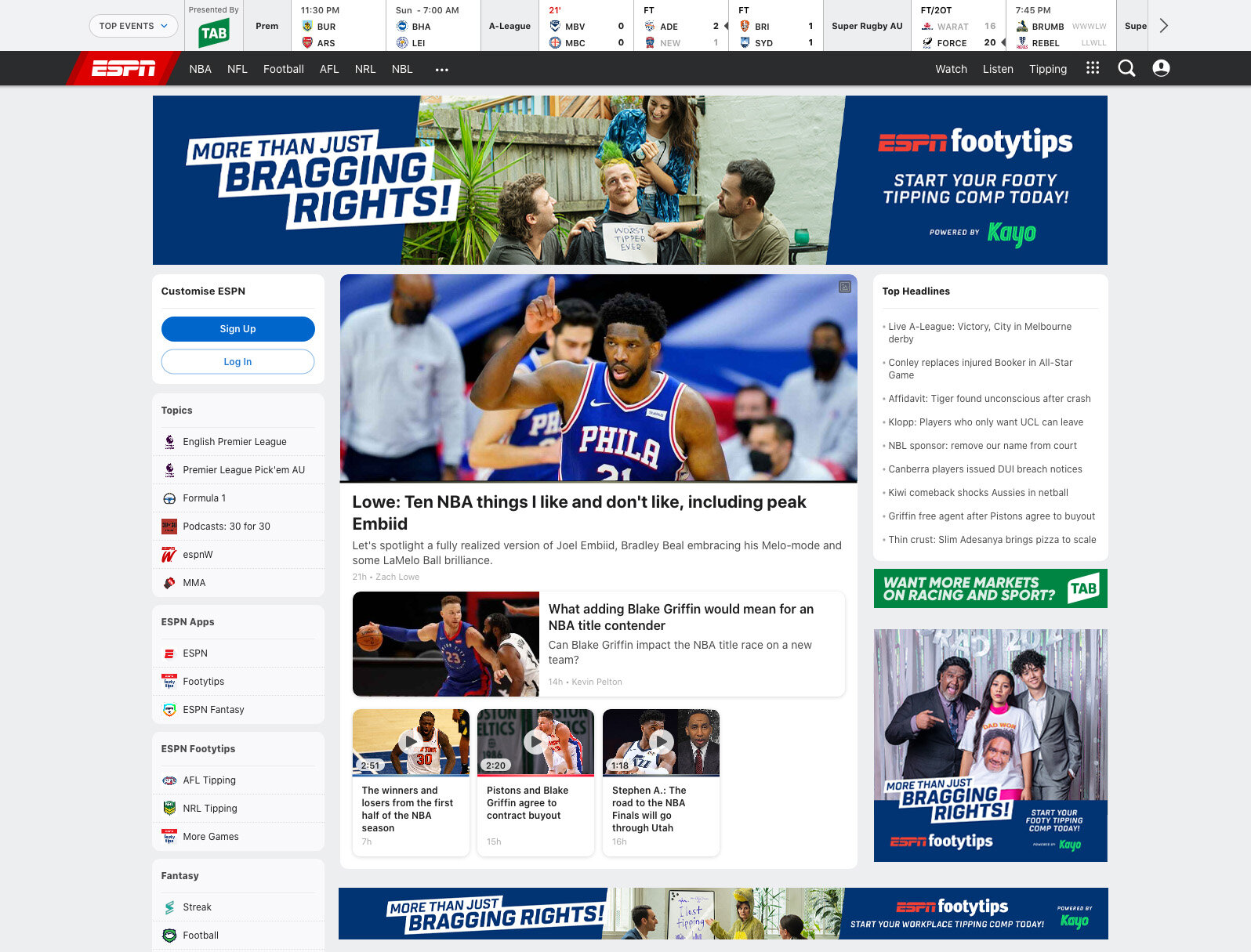Screenshot of ESPN Sports Dashboard

Background: Gray with highlights and various text overlays.

**Top Bar:** 
- "Top Events presented by TAB" (gray banner)
- "Premium Events" listing (11:30 PM: BUR vs. ARS, Sunday at 7:00 AM: BHA vs. LEI)
- Additional Scores:
  - MBV vs. MBC: 0-0 (FT)
  - ADE vs. NEW: 2-1 (FT, ADE in black, NEW in gray)
  - BRI vs. SYD: 1-1 (Super Rugby AU, FT)
  - WARAT: 16 vs. Force: 20 at 7:45 PM
  - BRUMB (WWWLLW) vs. REBELLLL

**Navigation Bar:**
- ESPN logo on the left, white text with a red diagonal box
- Categories: NBA, NFL, Football, AFL, NRL, NBL
- Additional Options: Watch, Listen, Tipping, Search, Account
- Grid of 9 dots for more options

**Advertisement Banner:**
- Featured ad for Kayo: "More than just bragging rights"
  - Theme: Two men labeling another man as "worst tipper ever" while a woman is shaving his hair
  - Message: "ESPN FTY Tips: Start your FTY tipping comp today, powered by Kayo"

**Left Sidebar:**
- Option to customize ESPN with blue "Sign Up" and "Login" buttons
- Topics List:
  - English Premier League
  - Premier League Pick'em
  - AU
  - Formula One
  - Podcasts
  - 30 for 30
  - ESPNW
  - MMA
- ESPN Apps and FTY Tips
- Games: AFL Tipping, NRL Tipping, More Games, Fantasy Box, Street Football

**Main Content:**
1. Article: "Low: 10 NBA things I like and don't like, including Peak EMBIID"
   - Description: Highlighting Joel Embiid, Bradley Beal, and LaMelo Ball
   - Image: Black player from the Philadelphia 76ers holding one finger up
2. Article: "What adding Blake Griffin would mean for an NBA title contender"
   - Inquiry: Blake Griffin's potential impact on the title race
   - Image: Griffin dribbling, holding off a defender
3. "The Winners and Losers from the First Half of the NBA Season"
4. "Pistons and Blake Griffin agree to contract buyout"
5. "Stephen A: The road to the NBA Finals will go through Utah"

**Right Sidebar Headlines:**
- Live A-League: Victory in Melbourne Derby
- Conley replaces injured Booker in All-Star Game
- Affidavit: Tiger Woods found unconscious after crash
- Klopp: Players who only want UCL can leave
- NBA Sponsor: Remove our name from court
- Canberra players issued DUI breach notices
- Kiwi comeback shocks offseason netball
- Griffin free agent after Pistons buyout
- DeCrossan, Adesanya brings pizza to scale

**Footer Advertisement:**
- "Want more markets on racing and sport?" in a green bar with tab logo
- Repeated ad for "ESPN Footy Tips: Start your footy tipping comp today"